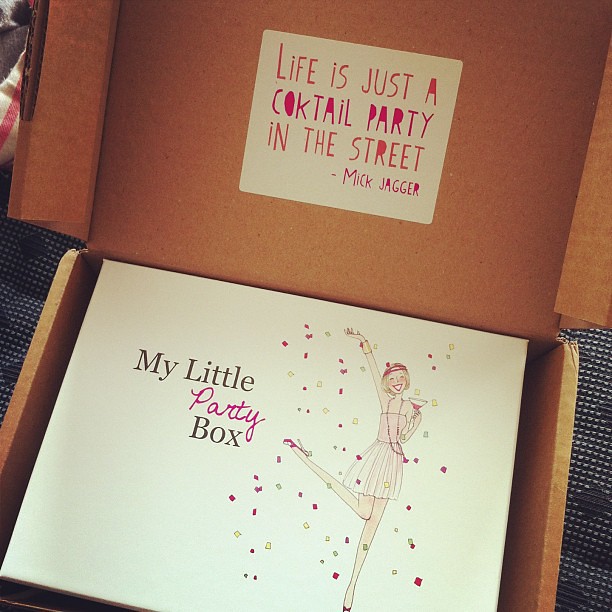A close-up photograph reveals an open cardboard box placed on a navy blue tablecloth, with a piece of white fabric featuring a red stripe in the top left corner. The lid of the cardboard box is folded up, displaying a piece of paper with pink text that reads, "Life is just a cocktail party in the street" attributed to Mick Jagger. Inside the cardboard box, there is another box labeled "My Little Party Box." This inner box, with a predominantly white design, features an illustration of a cartoon woman dressed in a bright pink top and lighter pink tutu. She has pink ballet shoes and is depicted with her left arm holding a martini glass filled with pink liquid. Her right arm is raised with her palm up, and her right knee is bent, creating an elegant pose. Surrounding the ballerina are colorful diamond-like stars in shades of pink, black, and yellow, as well as scattered confetti falling from above. The overall scene exudes a festive and whimsical atmosphere.